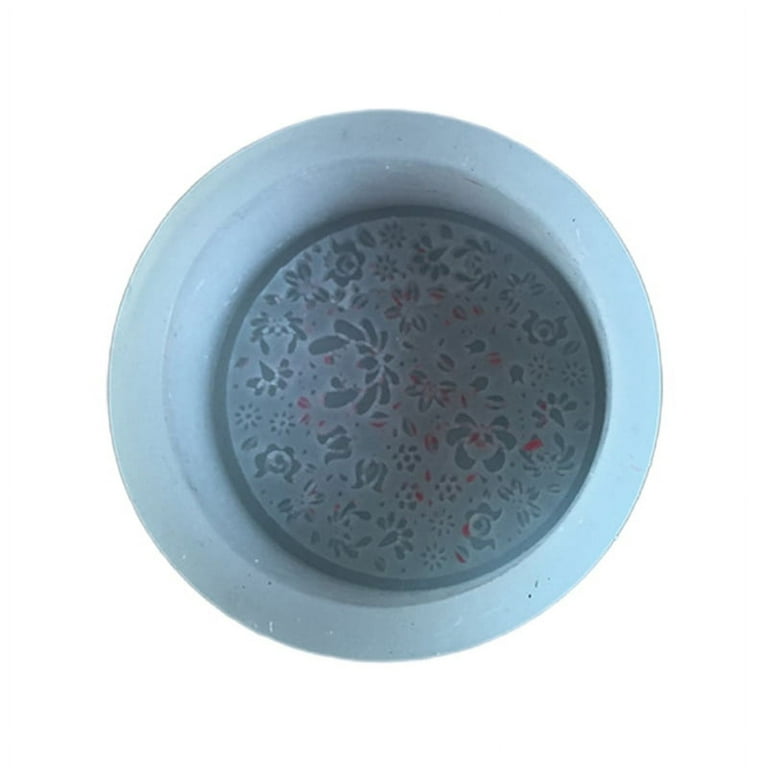The image depicts a top-down view of a small blue circular object resting against a pure white background. This object resembles a blue silicone mold or a plastic sink stopper. It features a flat outer rim of light blue, measuring about an inch to an inch and a half deep. Inside this rim, there's a circular design with a dark blue border and a medium gray background. The centerpiece is an intricate floral pattern comprising predominantly green hues with sparse red specks. The floral design is offset slightly to the right, enhancing the minimalistic, clean aesthetic of the image. The absence of text or additional objects emphasizes the central focus on the blue mold-like object floating on a pristine white backdrop.